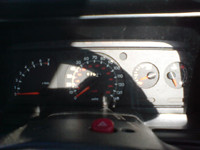A small-scale color photograph taken from the driver's point of view captures the car's dashboard and instrument cluster just beyond the top edge of the steering wheel. The image is saturated with heavy shadows, including those cast by the steering wheel and other interior elements. Visible in the shot is the top portion of the steering wheel and a conspicuous red button, likely the hazard light switch. 

Prominently featured in the instrument cluster are a tachometer and speedometer, both displaying red needles positioned at zero, indicating that the car is off. The speedometer has red markings with white numbers that are too small to read clearly. Flanking these primary gauges are two smaller meters, approximately a quarter to half the size of the main gauges, showing their lowest readings. These smaller meters are possibly for engine temperature and fuel levels. They also feature red or dark orange indicator arms against black backgrounds with white lettering, maintaining the consistent theme and color scheme of the dashboard instrumentation.